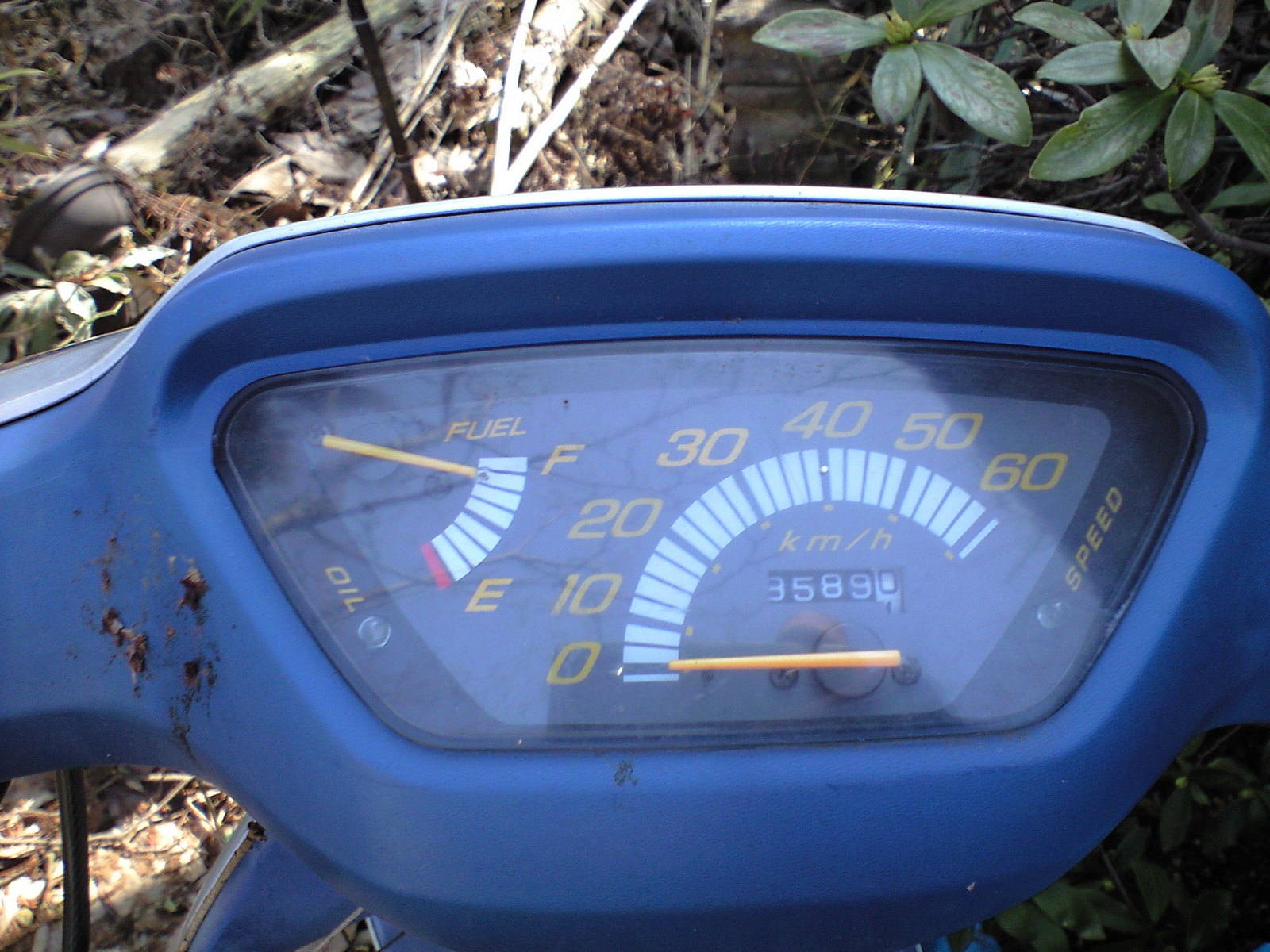The image showcases the front dashboard of a compact, motorized vehicle painted in a vivid blue color. Prominently displayed on the dashboard is a speedometer, with numbers ranging from 0 to 60 in yellow, complemented by a yellow needle indicating speed. Adjacent to the speedometer on the left is a fuel gauge marked "Fuel," displaying measurements from empty to full. Below the fuel gauge, there are labels indicating "Oil" on the left and "Speed" on the right. 

The background reveals a forested scene, with lush green leaves visible in the top right corner. Scattered around the dashboard are pieces of light brown wood debris, contributing to the natural, rugged environment. In the top left corner, a black, dome-shaped, rubbery object is partially visible, adding to the context of an outdoor setting.